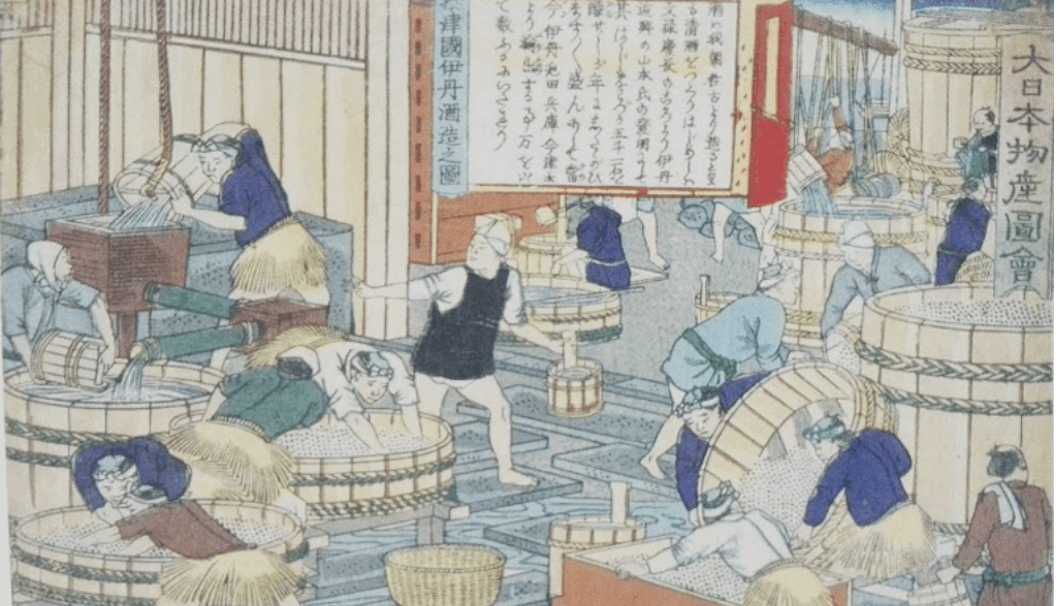This vintage, hand-drawn image depicts approximately 30 workers in a traditional Asian washhouse or factory, characterized by its muted yet intricate color palette. The scene is filled with individuals, most donning either bright or pale blue shirts tied around the waist with sashes, and some sporting grass-like skirts reminiscent of the wicker baskets they're using. Their skin tones are off-white and their facial features are simplistic. They are engaged in various tasks around large circular wooden bins, some sifting through materials, while others scoop and pour water into containers. Notable details include a worker to the left pouring water into a large box connected by green pipes and hoses, and a central figure clad in a black vest over a long-sleeved white shirt, short white shorts, and a towel atop his head.

The backdrop is rich with Asian textual elements: a white square with Japanese hiragana characters, a blue rectangle with Chinese characters or kanji, and a banner on the right side with additional Japanese text. The floor is blue with a pattern of rectangles, adorned with various old washing machine devices. The overall slightly yellowed appearance of the image adds to its aged charm.